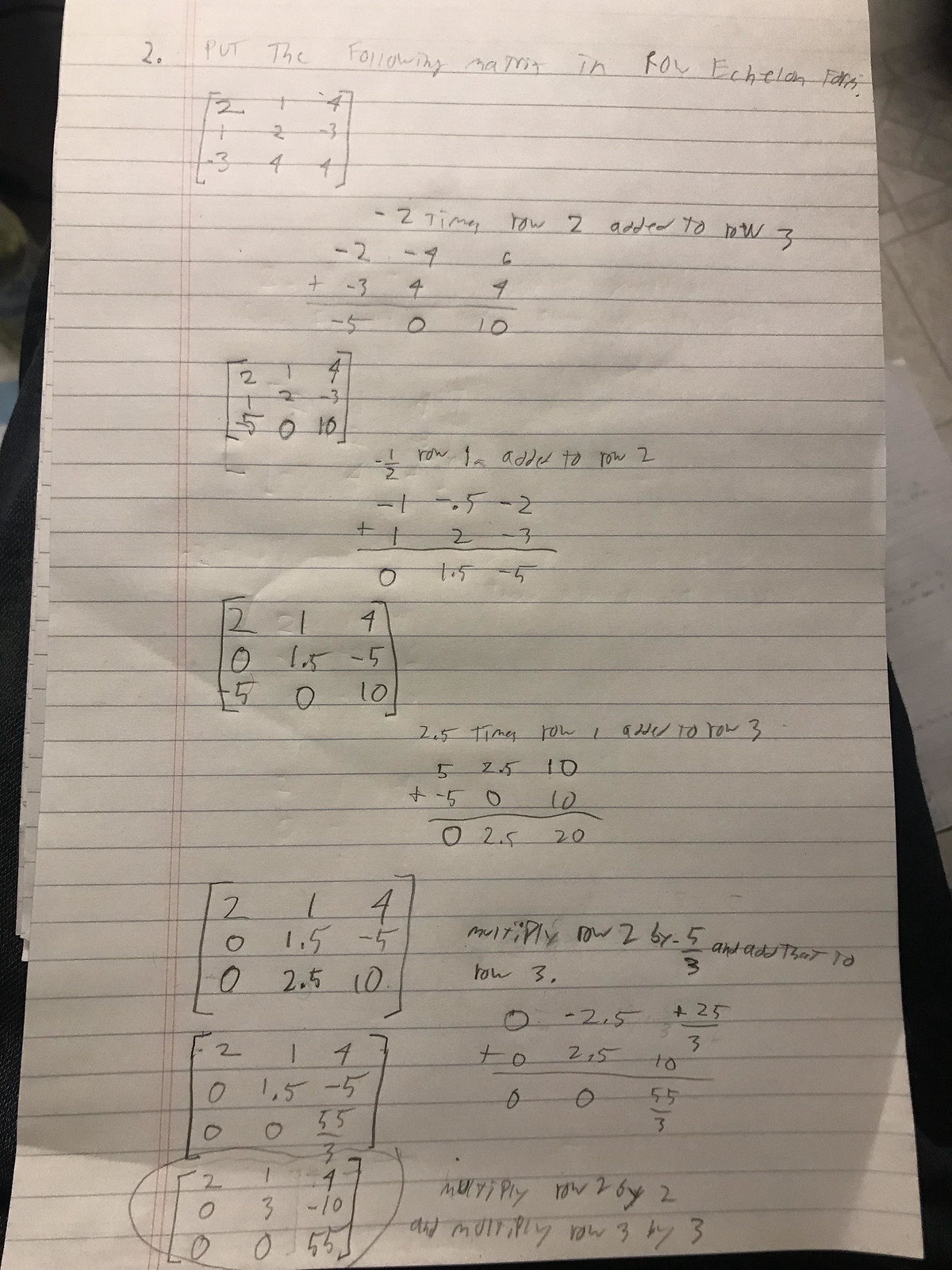The image features a piece of lined paper from a pad, displaying a single, detailed mathematics problem. The problem is worked out step-by-step, with each stage of the solution meticulously handwritten. The paper, characterized by its wide spacing, is divided into six distinct sections, guiding the reader through the logical progression of the problem. The final answer is prominently circled at the bottom left of the sheet. On the left-hand margin, plot points are enclosed in brackets, while the corresponding calculations occupy the right-hand side. The background reveals a tan-tiled floor, and a second pad is visible, partially obscured by the person's leg, indicating that the paper comes from several pages into the pad. The mathematical content suggests the problem may involve graphs or calculus, emphasizing the methodical nature of the solution process.